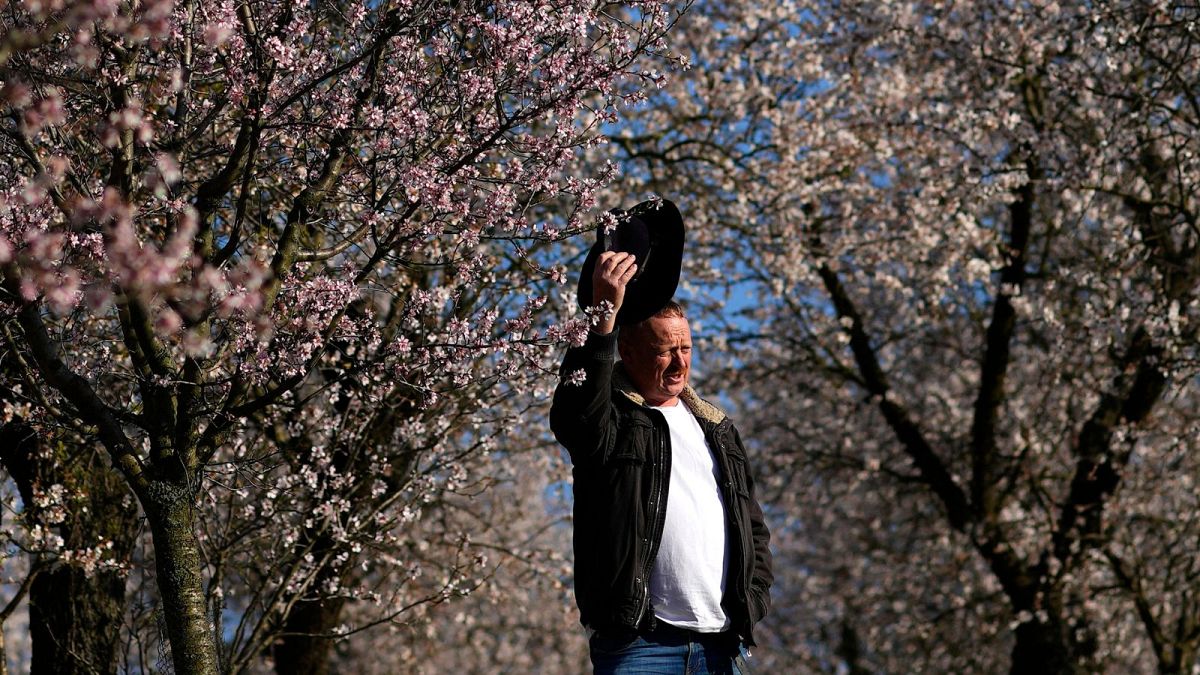This color photograph captures the serene beauty of a blooming cherry blossom landscape. Dominating the background are brown-branched trees densely covered with small pink and white blossoms, creating a lush canopy that nearly obscures the blue sky. In the middle of this picturesque scene stands an older Caucasian man with ginger hair. He wears a black jacket with a tan collar over a white t-shirt and blue jeans. His round stomach is noticeable under his shirt. With one hand, he holds a lifted black cowboy hat, suggesting he has just removed it, possibly due to the warm weather. He squints slightly while looking off to the right, his face revealing a few forehead wrinkles. His other hand rests in his pocket, contributing to a relaxed posture. The man's sideways gaze and the natural setting evoke a moment of quiet reflection amidst the blooming cherry blossoms.